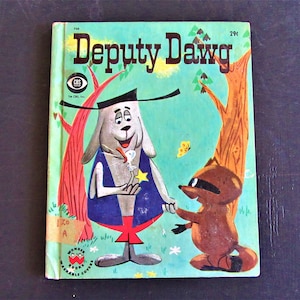The photograph features a vintage children's book titled "Deputy Dog," set against a bluish dark background. The cover, rendered in a light turquoise blue, showcases a charming scene reminiscent of 1940s and 1950s artwork. At the center, a rotund dog, bearing a resemblance to the Looney Tunes character Droopy in the face, stands with droopy eyes and a wide-brimmed hat adorned with a star badge. In his right hand, he holds a small bird, while his left hand warmly clasps that of a raccoon. The backdrop includes two brown-trunked trees with small green leaves, and a couple of butterflies fluttering near the characters. Above the scene, the title "Deputy Dog" is prominently displayed in black lettering. The cover also features various emblems, with one resembling an eye and another, indistinct red stamp, located in the bottom left corner.